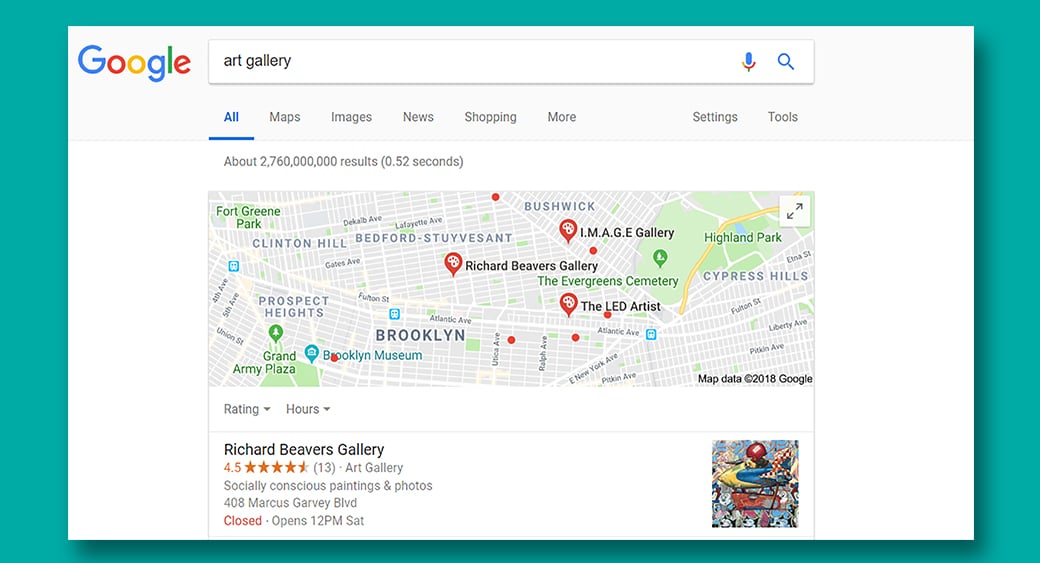In this image, a Google search page displays results for "research interviews at the Gallery." The search yields approximately 2,760,000,000 results in 0.52 seconds. The page features various search categories including Maps, Images, News, Shopping, More, Settings, and Tools. 

Below these categories, a map pinpoints several locations in Brooklyn, New York. The highlighted areas include Fort Greene Park, Clinton Hill, Bedford-Stuyvesant, Prospect Heights, Grand Army Plaza, Brooklyn Museum, Richard Beavers Gallery, The Evergreen Cemetery, Highland Park, Cypress Hills, Fulton Street, E. New York Avenue, Pitkin Avenue, and Atlantic Avenue. 

A specific entry on Richard Beavers Gallery is marked, featuring its 4.5-star rating garnered from 13 reviews. This detailed overlay provides a concise yet comprehensive snapshot of the searched topic with relevant geographic and evaluative information.